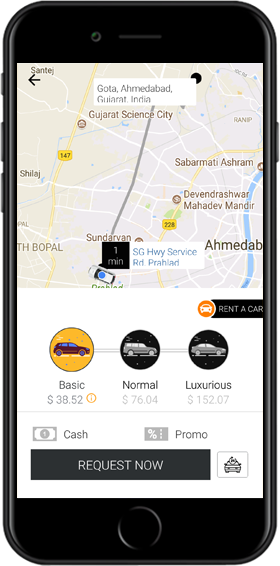In the image, a smartphone is prominently displayed against a plain white background. The device appears compact compared to modern smartphones. It features a small speaker and a camera just above the screen. On the left side of the phone, there is a small button and two slightly larger buttons, possibly for volume control. The right side of the phone has a singular medium-sized button.

The screen shows a navigation application, likely an Uber app. The map highlights various roads, including routes 147 and 228, running vertically. Several cities are listed, such as Santaj, Shilaj, Sundarvan, Sabarmati Ashram, and Gujarat Science City. The destination on the screen is Gota in Ahmedabad, Gujarat, India. A navigational line extends from a car icon to a black dot indicating the destination. Different fare options are shown: Basic at 38.52, Normal at 76.04, and Luxurious at 152.07. At the bottom of the screen, the option to "Request now" is visible.